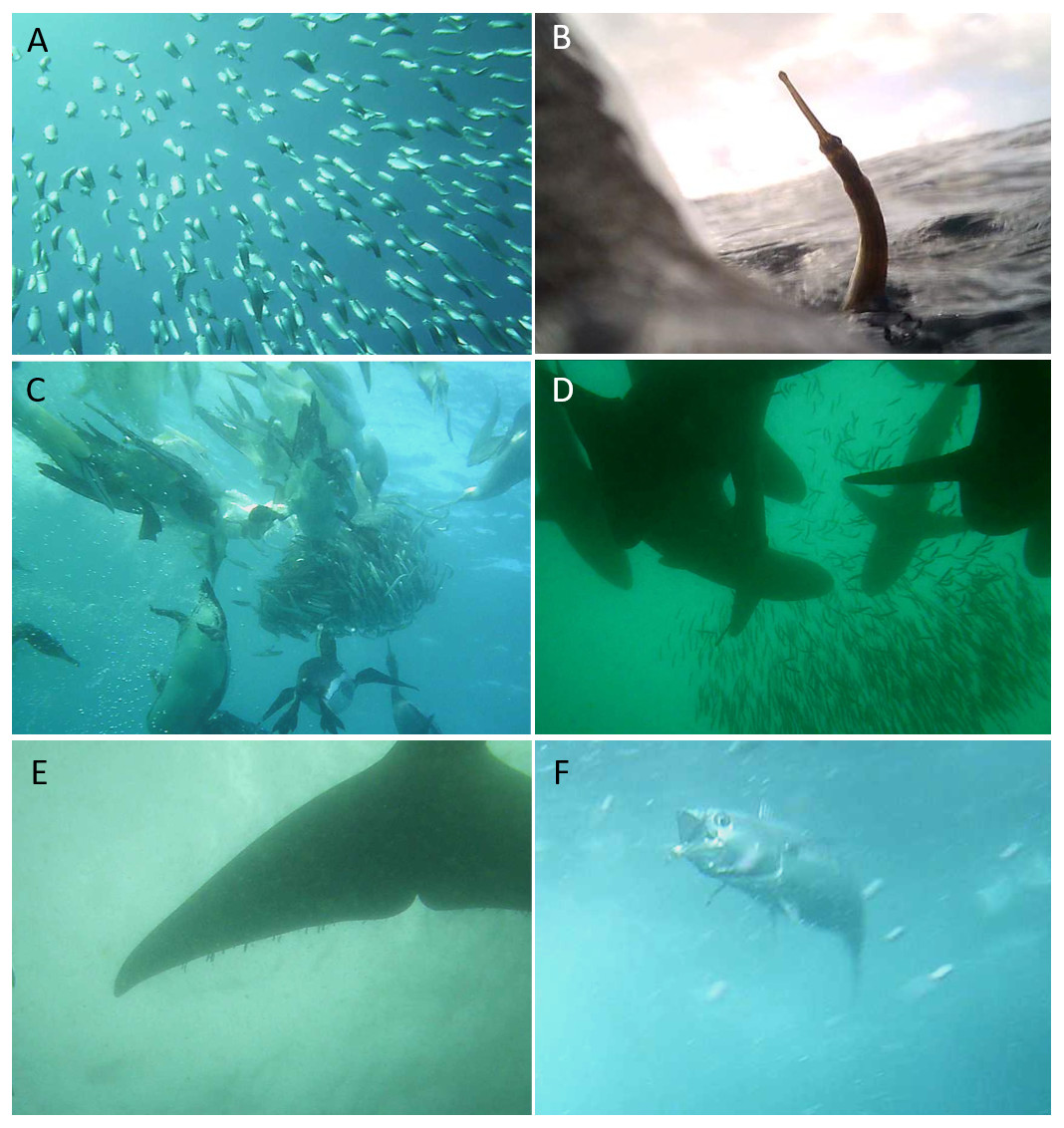This collection features six vibrant, labeled photographs (A through F) of diverse oceanic scenes, predominantly underwater. 

Photo A presents a dynamic school of tiny fish swimming in formation. 

Photo B displays a peculiar, possibly computer-generated, curved cylinder with an extending tentacle or appendage emerging from the water's surface.

Photo C captures numerous larger fish gliding through serene blue waters.

In Photo D, the silhouettes of hammerhead or possibly other shark species can be seen navigating through greenish waters, accompanied by another school of small fish.

Photo E showcases the impressive tail of a large marine animal, likely a whale, emphasizing the enormity and grace of these creatures.

Finally, Photo F features a detailed image of a large fish with its mouth open, set against more blue water, highlighting the intriguing marine life within these varied ocean hues.